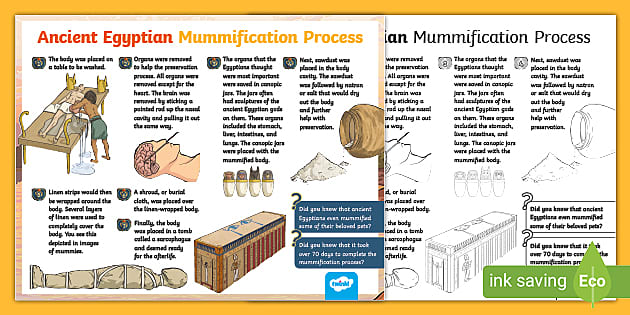This detailed poster illustrates the ancient Egyptian mummification process in a step-by-step format, complete with descriptive text elevating the educational content. The diagram features a series of stages, beginning with an image of a person laying down, and visually walks the viewer through various procedures such as draining bodily fluids and extracting the brain. The mummified remains are shown in characteristic containers, leading up to the final depiction of the mummy and its tomb. The poster is presented twice: once in full color with a vibrant palette of red, yellow, and green on a yellow background, and once in a black-and-white, ink-saving version. The black-and-white version is marked with a green banner in the lower right-hand corner, within which a teardrop-shaped icon touts "ink-saving eco," emphasizing its economy-friendly design. Despite its dual presentation, the contents and instructional value remain consistent, serving as a captivating and informative resource on ancient Egyptian burial practices.